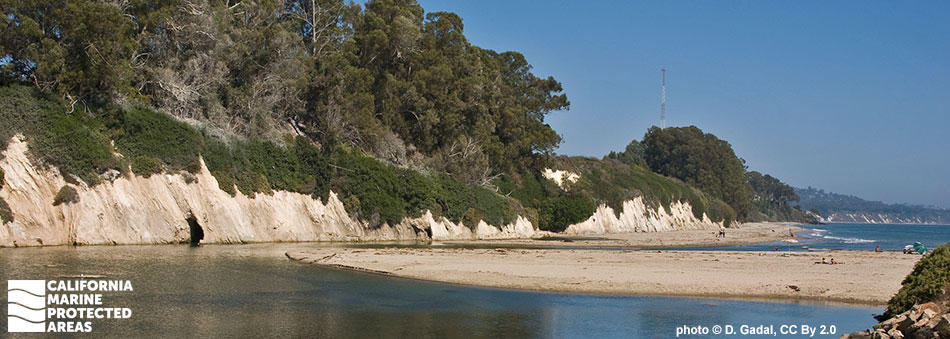This landscape photograph of the California coast, titled "California Marine Protected Areas," is nearly three times wider than it is tall and vividly captures the serene coastal environment. The bottom left corner features a rectangular design with wavy lines and the text "California Marine Protected Areas," while the bottom right corner shows "Photo © d.getal, CC BY 2.0."

In the foreground, the picture showcases a mixture of green and brown waters on the left, transitioning to a clearer blue on the right. A rocky incline with dark green plants and eucalyptus trees extends from the bottom left to the top of the image, where it meets more bluffs adorned with vegetation. The immediate coastal area includes a sandbar and a potential beach or walkway, adding layers to the landscape.

Further back, the scene reveals additional water bodies and beaches, framed by distant hills and mountains. You might notice a red and white telephone tower subtly integrated into the distant horizon, adding a modern touch to the natural scenery. Small details like a beach umbrella and a few barely discernible people resting on the sandbar enrich the scene's liveliness, offering a glimpse into human interaction with this protected marine area.